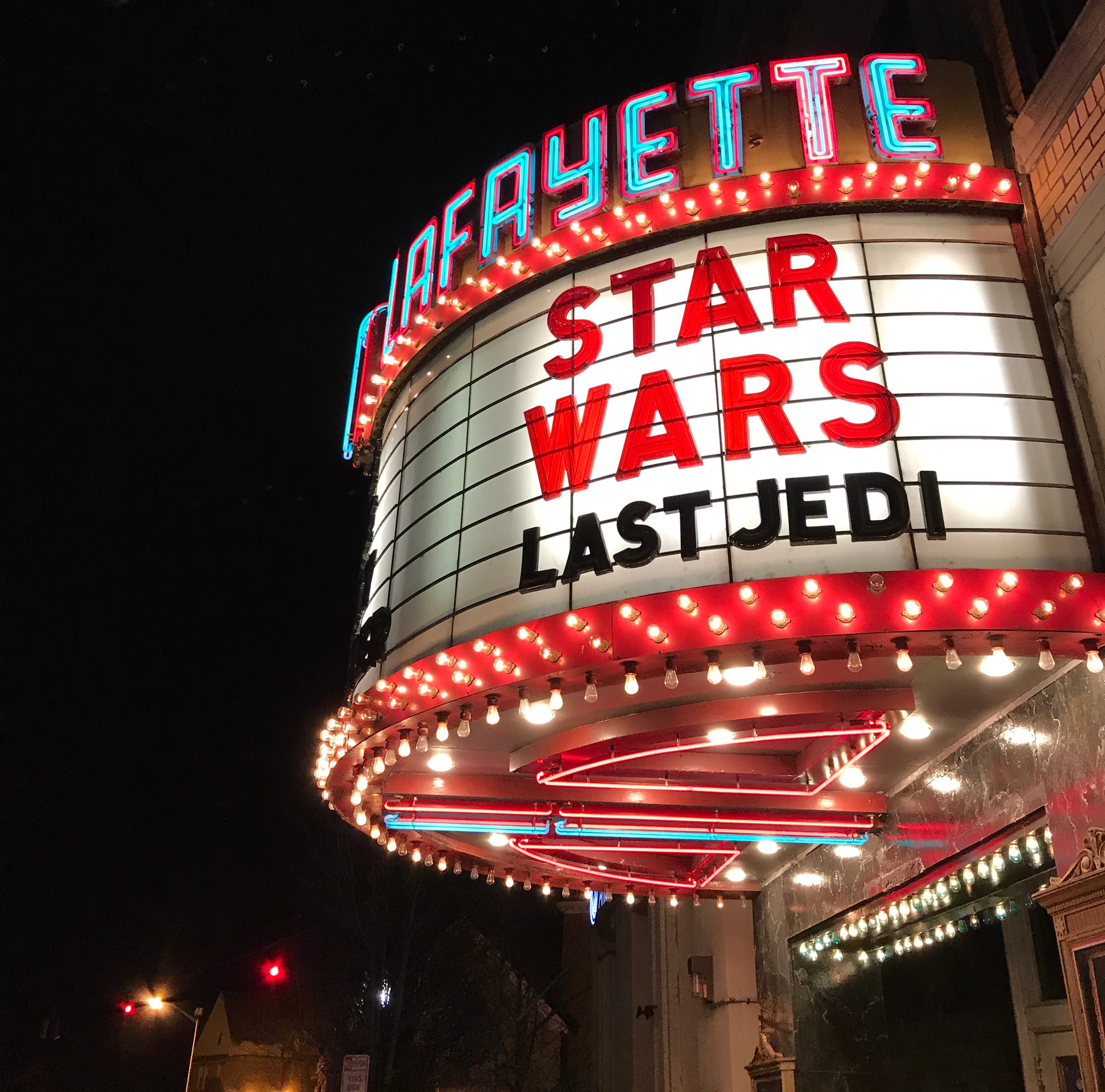This vibrant, vertically rectangular, nighttime photograph captures an old retro 1950s-style movie theater marquee. The sign, vividly illuminated against a black sky, displays "Lafayette" in electric blue and red neon lights, with a red border lined with white lights. Below, a white background with plastic lettering reads "Star Wars" in red and "Last Jedi" in black, enclosed by another red, light-covered border. To the lower-left corner, off in the distance, a stoplight and street sign can be seen near a house. On the right side, the marquee dominates the scene, attached to a white-walled building. The entrance of the theater, just visible beneath the marquee, showcases a cool design typical of the era, reflecting the craft and style of the times. Overall, the photo's bright, colorful elements of red, white, yellow, and blue lights bring the marquee to life, contrasting beautifully with the night sky.